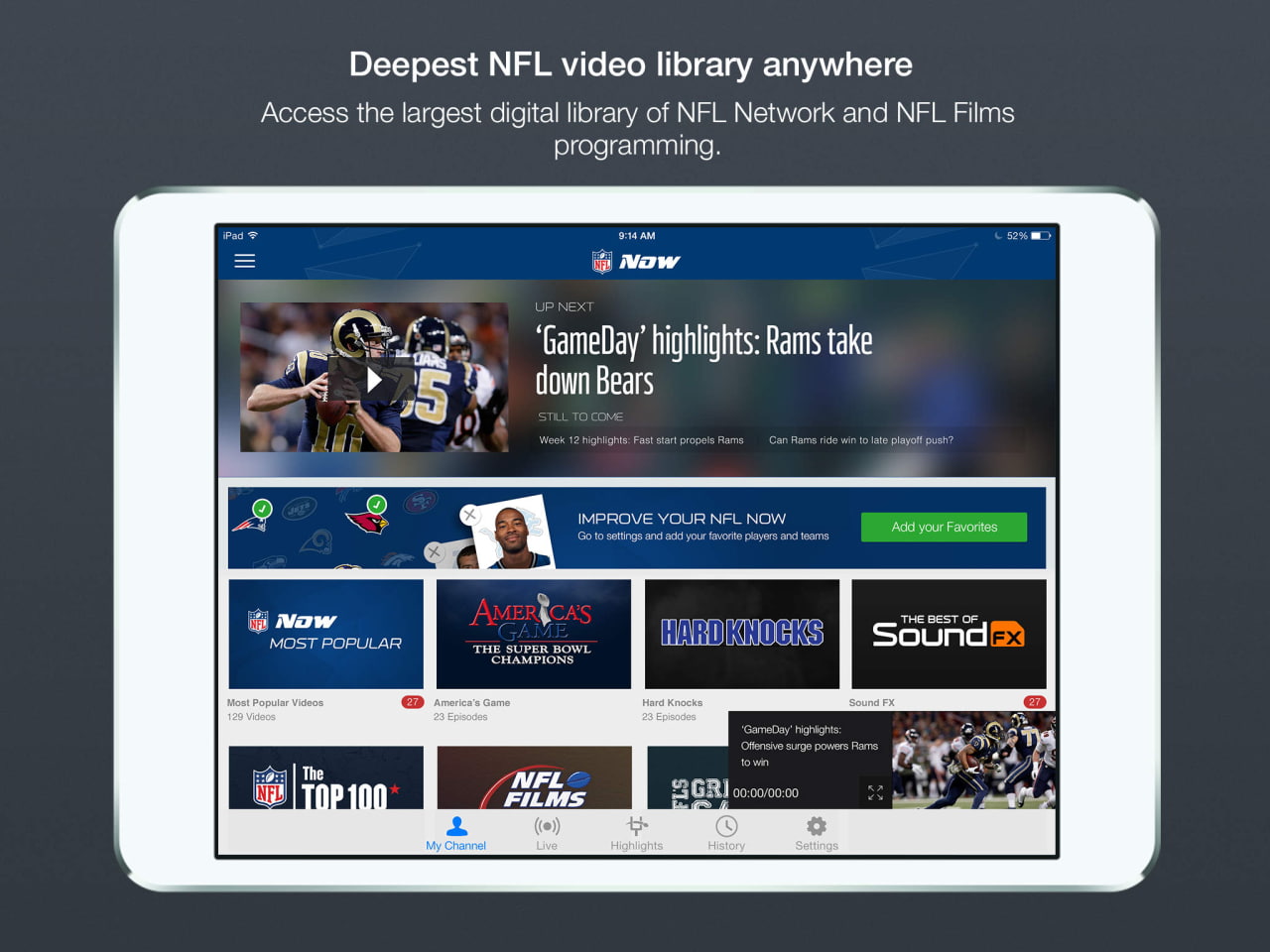The photo features an advertisement for an NFL-focused app, meticulously detailed in a landscape-oriented, rectangular image. Set against a gray background, the center showcases an illustrated iPad-like device, potentially sketched with a superimposed screen display.

At the very top center of the photo, bold white text proclaims, "Deepest NFL Video Library Anywhere." Directly beneath this, it reads, "Access to the Largest Digital Library of NFL Network and NFL Films Programming." 

Below these headings, the illustrated iPad device with a gray edge and an inner white border takes focus. The screen displays a detailed interface, beginning with a blue banner showing standard iPad indicators: a Wi-Fi connection icon, a moon icon, and a battery indicator showing 52% charge.

The banner also bears the app's name, "NFL Now," followed by visual content. Prominently featured is a game-day highlight image of a St. Louis Rams player, accompanied by text stating, "Game Day Highlights, Rams take down Bears."

Below this, another blue box presents images of the New England Patriots and the Arizona Cardinals, alongside the text, "Improve your NFL Now, add to your favorites." 

Further down, the interface includes a row of clickable thumbnails with titles such as "Most Popular Videos," "America's Game," "Hard Knocks," "Best of Sound FX," "NFL Top 100," and "NFL Films," though some items are cut off from view. 

This comprehensive layout effectively markets the extensive video library and interactive features available through the NFL Now app, appealing to dedicated football enthusiasts.